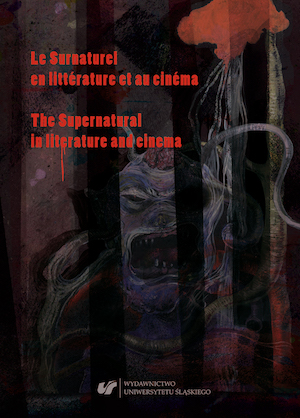This is a dark-themed, square-shaped poster for a supernatural-themed cinematic event or film. The poster prominently features an eerie, ghostly alien figure with only its head visible, which has partially formed teeth. The alien appears to be trapped behind bars, adding to the sinister feel of the image. Written across the top in bold red text are the words "Les Surnaturelles en Littérature et au Cinéma," which translates to "The Supernatural in Literature and Cinema." Below this, the translation is repeated in English, also in red. At the bottom center of the poster, the name "Wendat Tigtel" and a logo for the University of Slaskago can be seen, indicating the institution associated with the event. The primary colors of the poster are black and red, with the alien figure rendered in white and red, enhancing the spooky, dark aesthetic.